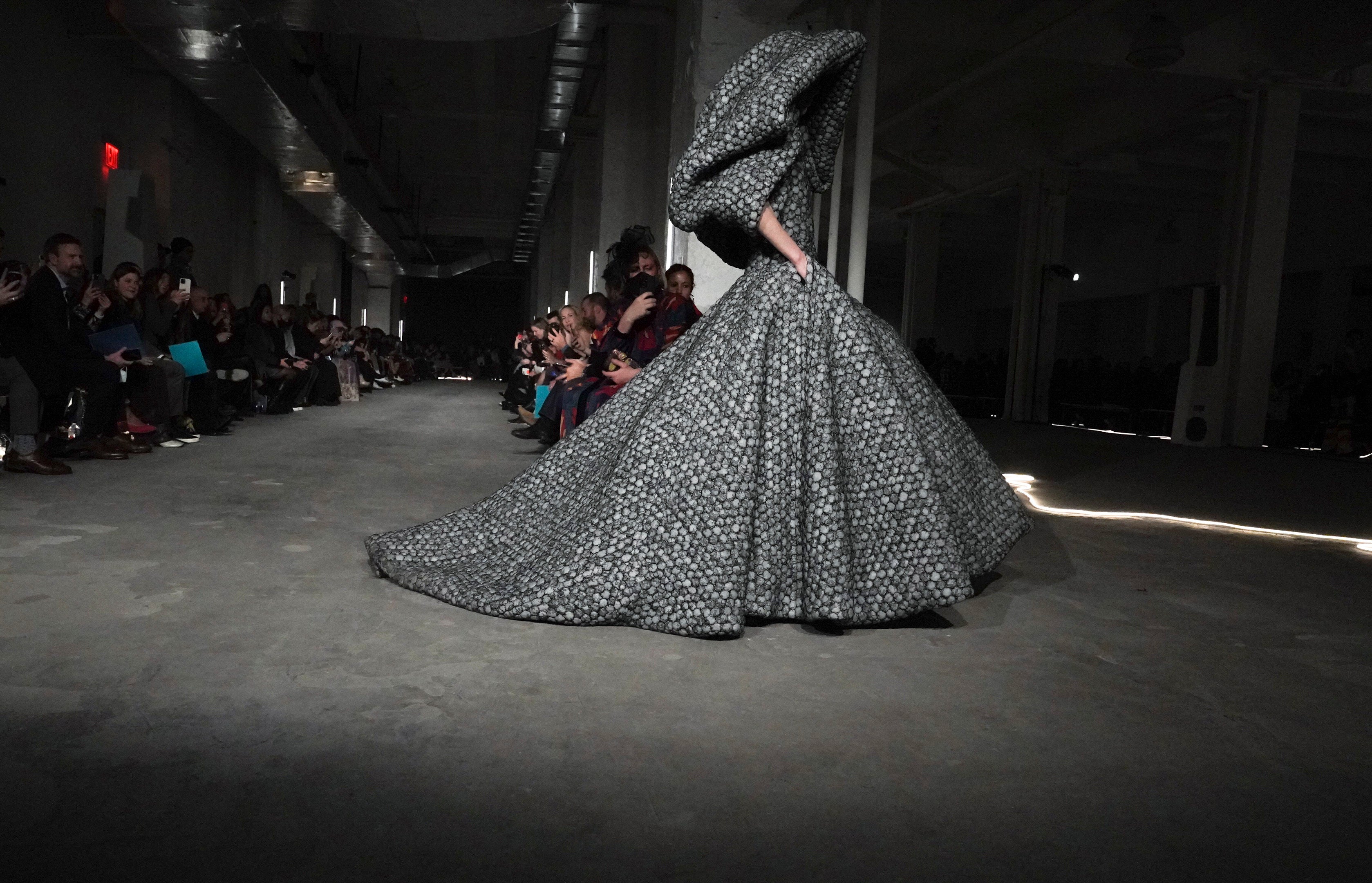This detailed photograph captures the dramatic moment at a fashion show, likely held in Milan or Paris during the fall or winter season. The event takes place in a dimly lit, industrial warehouse with dark gray floors and structural pillars adding to the ambiance. The long runway stretches between rows of seated audience members who are engrossed in capturing the spectacle with their phone cameras. The model, having just completed her walk, is turning, stepping from the runway into another dimly lit area of the venue. She is adorned in an eye-catching, monochromatic ensemble—a gray, three-quarter sleeve, hooded dress that boasts an enormous, trailing train. The hood is oversized, completely covering her face and lending an air of mystery, while only her right arm, from elbow to wrist, is visible, as her hand rests in a pocket. The dress, made to make a striking visual impact, is polka-dotted in gray, enhancing its dramatic effect against the dark backdrop. The photograph captures the elegant yet industrial essence of this high-fashion scene.